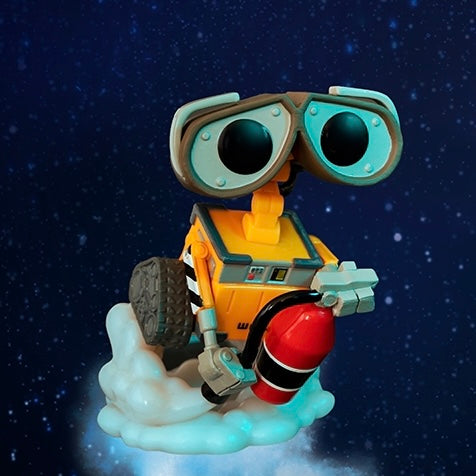The image depicts a toy robot with a golden-yellow square body and a single black tire on its side. The robot has small yellow arms, one of which holds a black and white sign. In front of the robot is a red fire extinguisher connected to a gray hose, which attaches to the robot's gray hands extending from its yellow torso. The robot appears to be equipped with a scuba tank-like apparatus. Its head features a pair of goggles, with a dark gray trim and light gray centers highlighted by large black circular eyes, evoking the appearance of underwater diving gear. The scene is set against a navy blue background adorned with tiny white specks, reminiscent of a starry night sky. At the bottom, there are white elements resembling clouds, adding to the whimsical and imaginative atmosphere.